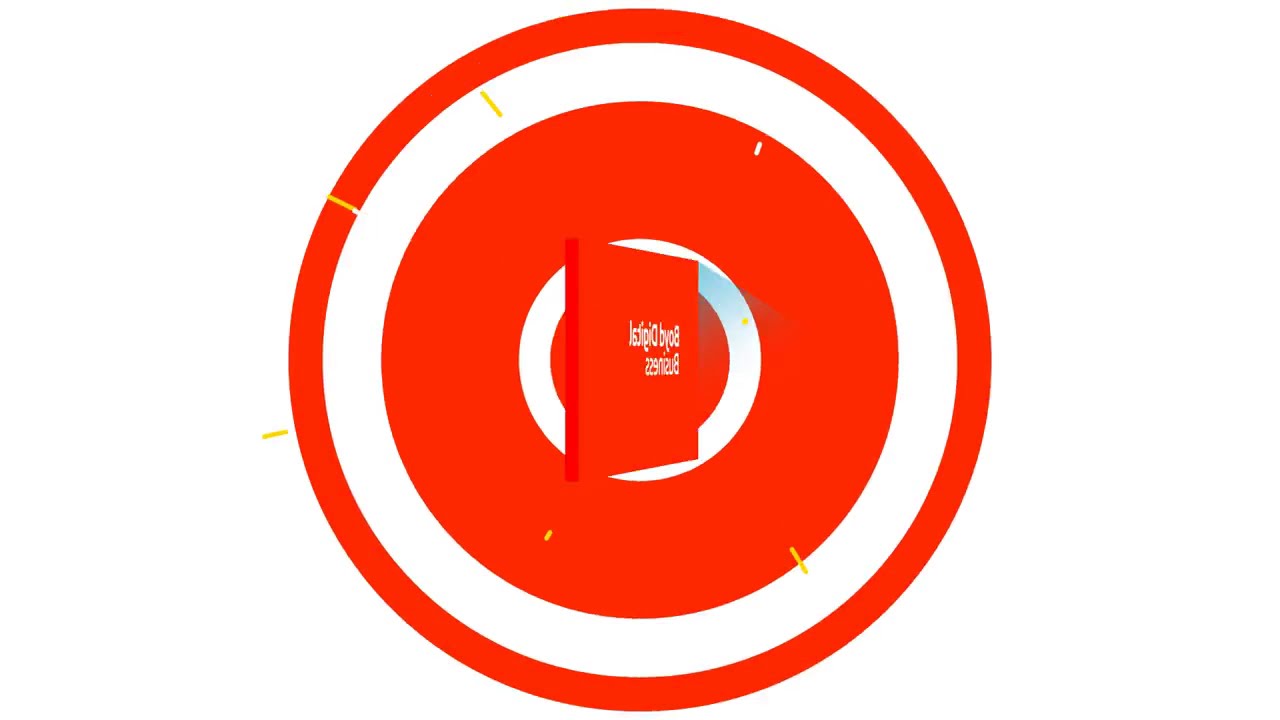The image features a pure white background with a striking, centrally placed red bull's-eye comprised of concentric rings. These rings alternate between red and white, starting with a thin red outer ring followed by a slightly wider white ring. The sequence then presents a much wider red ring, a thin white ring, and culminates in a solid red central disc. Hovering above this central disc is a slightly rotated rectangular object bearing white text on two lines, which appears difficult to read as the characters are flipped. Among the letters, potential fragments include 'B', '0', 'I', 'S', and '8'. Scattered across various parts of the bull's-eye are random yellow markings, with one notable marking positioned completely outside the disc on the left side. These yellow bars or lines add an element of curiosity, possibly indicating some form of impact or annotation. The overall composition exudes a graphical and somewhat three-dimensional design with intriguing textual elements.